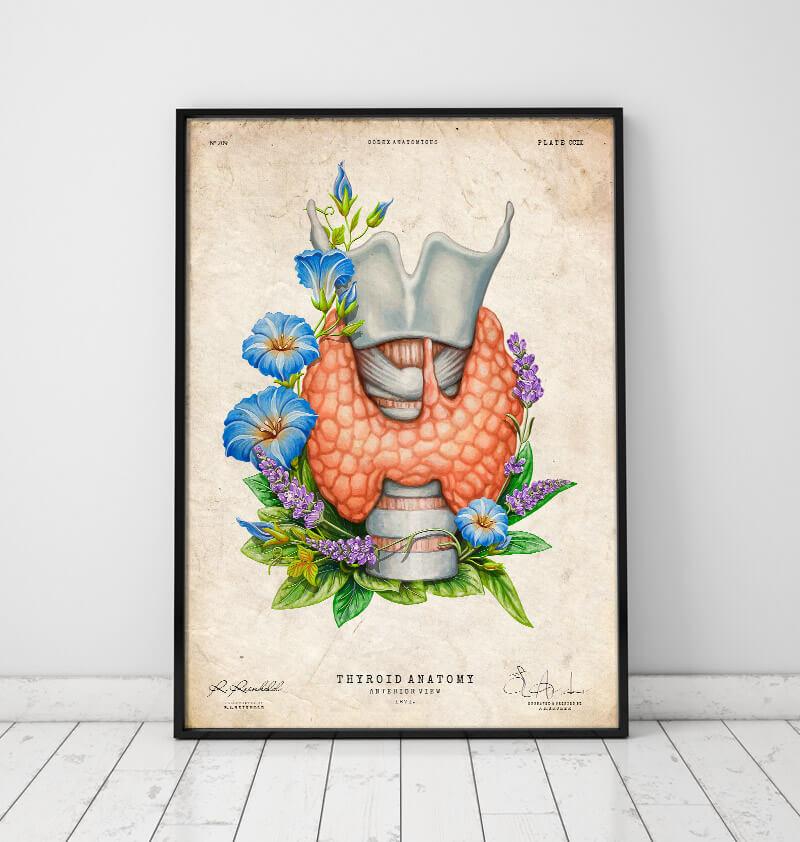The image features a framed art print titled "Thyroid Anatomy," depicting the front skeletal and muscle view of a human thyroid. The artwork is elegantly intertwined with purple lavender flowers, vibrant blue and white morning glories, and lush green leaves, creating a striking and artistic representation. The background appears as a parchment-style light brown, adding a vintage feel to the piece. The print is set within a thin black frame, which leans against a white wall with wooden trim and rests on a wooden floor, enhancing its rustic charm. The caption "Thyroid Anatomy, Interior View" is displayed prominently at the bottom in black print, flanked by signatures on both the left and right sides, further adding to its detailed authenticity.